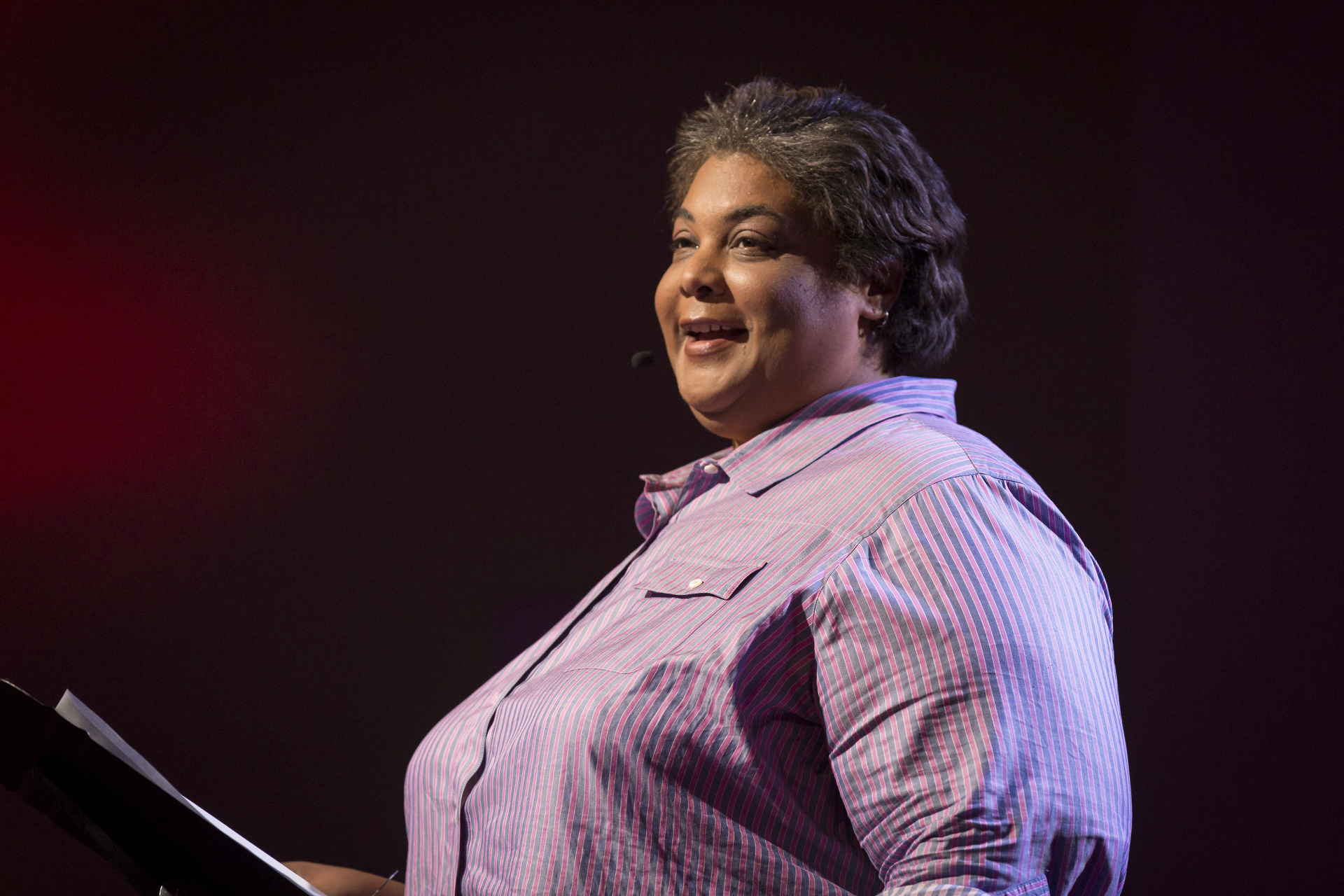The photograph captures a woman mid-presentation, illuminated by a bright spotlight that suggests an indoor, staged setting. She is standing behind a podium that has papers on it, reinforcing the idea that she is actively engaged in delivering a talk. Her body is facing to the left, presenting her side profile to the camera.

She has light brown skin and short, wavy hair that is predominantly black with a sprinkling of gray at the front—a "salt and pepper" appearance. She is wearing a lightweight, long-sleeved, button-down shirt adorned with vertical stripes in pink, blue, and white. There is a pocket on the left side of her chest, which features a buttoned flap. Complementing her attire, she wears minimal jewelry, limited to possibly small earrings.

A headpiece microphone is positioned near her mouth on the right side, indicating her active engagement in speaking. Her facial expression is friendly and approachable, with a genuine smile and dark brown eyes that suggest a pleasant demeanor. The background of the image transitions from black on the right to reddish tones on the left, remaining largely indistinct and blurry to keep the focus squarely on her.